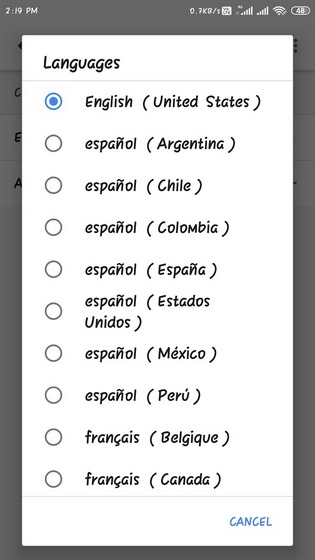The image displays an interface on what appears to be a digital screen. At the top, there is a light to medium gray rectangular area showing "2:19 PM." To the right of this, some text is partially obscured and illegible. Below, there is a white square with gray text inside it, but its contents are not discernible. Following this, a series of vertical lines increase in height from left to right, repeating this pattern again. Adjacent, there is a Wi-Fi symbol and an oval containing the number "48."

Beneath this, a prominently displayed white rectangle has "Languages" written at the top in bold. Inside, the first option displayed is "English" followed by "(United States)" in parentheses, accompanied on the left by a blue circle with a blue outline, indicating selection. Below, there are several language options each paired with a corresponding country in parentheses and a gray outline circle to their left: 

- "Español" (Argentina)
- "Español" (Chile)
- "Español" (Colombia)
- "Español" (España)
- "Español" (Estados Unidos)
- "Español" (Mexico)
- "Español" (Peru)
- "Français" (Belgique)
- "Français" (Canada)

At the very bottom of the interface, there is a blue button labeled "Cancel."